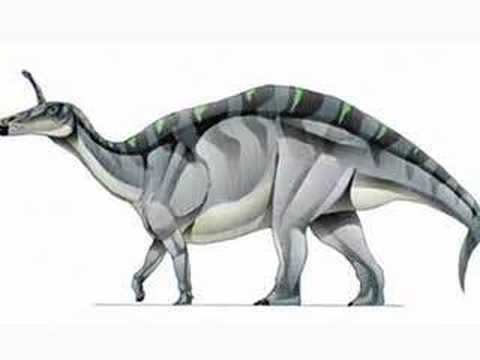This image is a detailed drawing of a dinosaur rendered in black and white with hints of color, featuring no background or border. The dinosaur is in a left-facing profile, showcasing its distinctive features. It has four legs, with the back legs significantly thicker and more muscular than the shorter front legs, akin to a T-Rex's posture. The skin texture displays varied shades of gray, and there's a notable fan-like structure on its back with a patterned mix of gray, black, and subtle green tones. This creature sports a singular horn protruding from its forehead, resembling a telescope. Its tail is long, though not excessively so. The underbelly is white, contrasting with the gray and black-striped sides, and the top exhibits a greenish hue. While the illustration captures some realistic elements, the design seems to blend fantastical aspects, leaving ambiguity about whether it represents a specific dinosaur species or a creative interpretation.